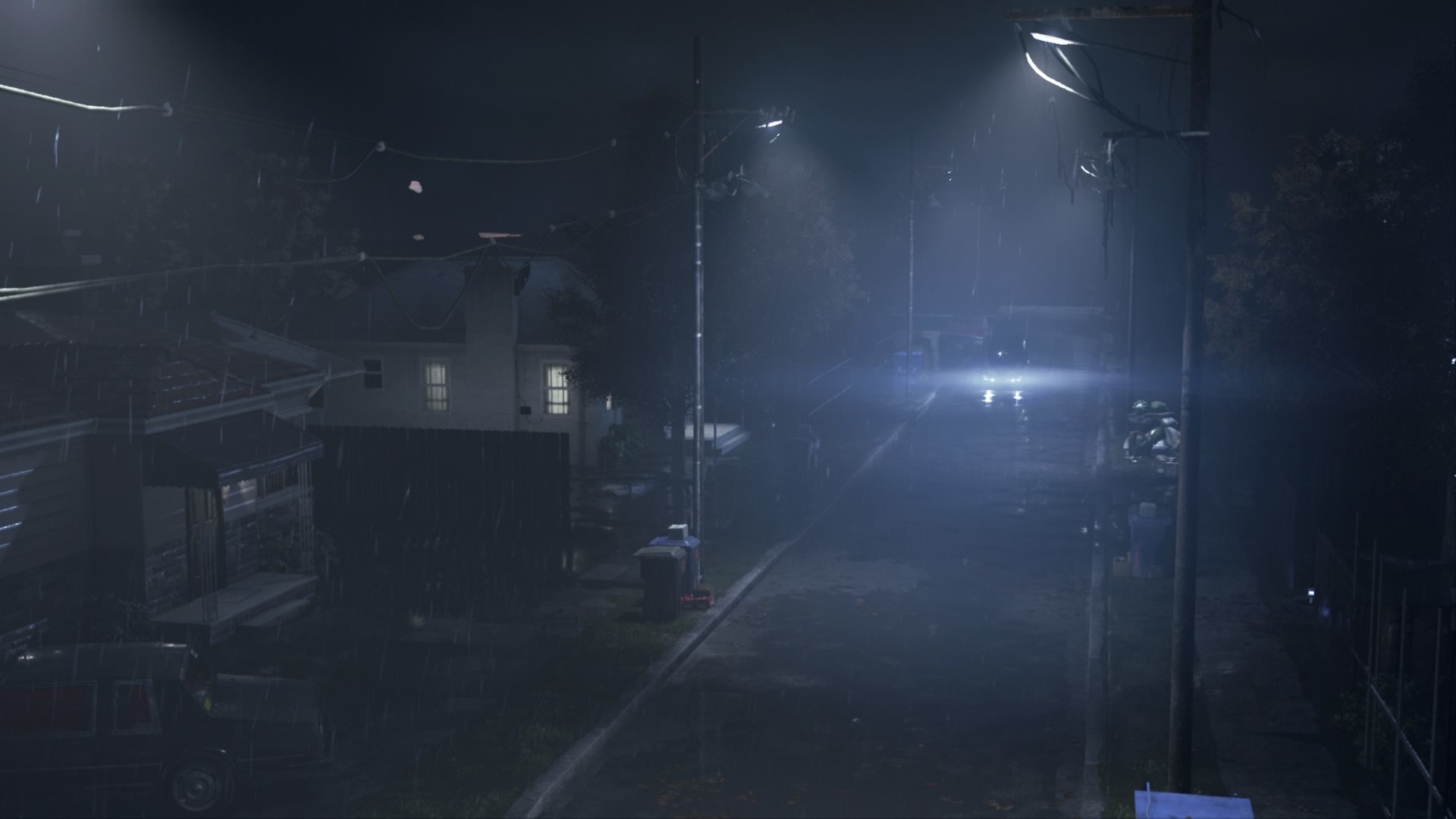This is a dark, night-time colour photograph taken from an elevated perspective, featuring a predominantly black and blue colour palette. The scene is a somewhat desolate streetscape with a single car approaching in the distance, its headlights diffusing through a light mist, suggesting either fog or rain. The limited street illumination and scattered glow from various sources give the scene a gloomy atmosphere. 

To the left, there's a series of buildings starting with a single-family home with a porch, next to which stands a tall picket fence beside trash cans, one regular and one for recycling. Adjacent to the picket fence is a white two-story house with lights visible in the windows, indicating some signs of habitation. In front of this house, an older model gray Cadillac is parked. The streetscape also features telephone poles and wires stretching across the scene, adding to the urban atmosphere.

On the right-hand side, a sidewalk runs parallel to the metal fencing or gate, contributing to the distinct division between public and private space. The combination of dim streetlights and the wet-looking street surface, possibly hinting at recent rainfall, completes this scene that blends realism with an air of mystery.